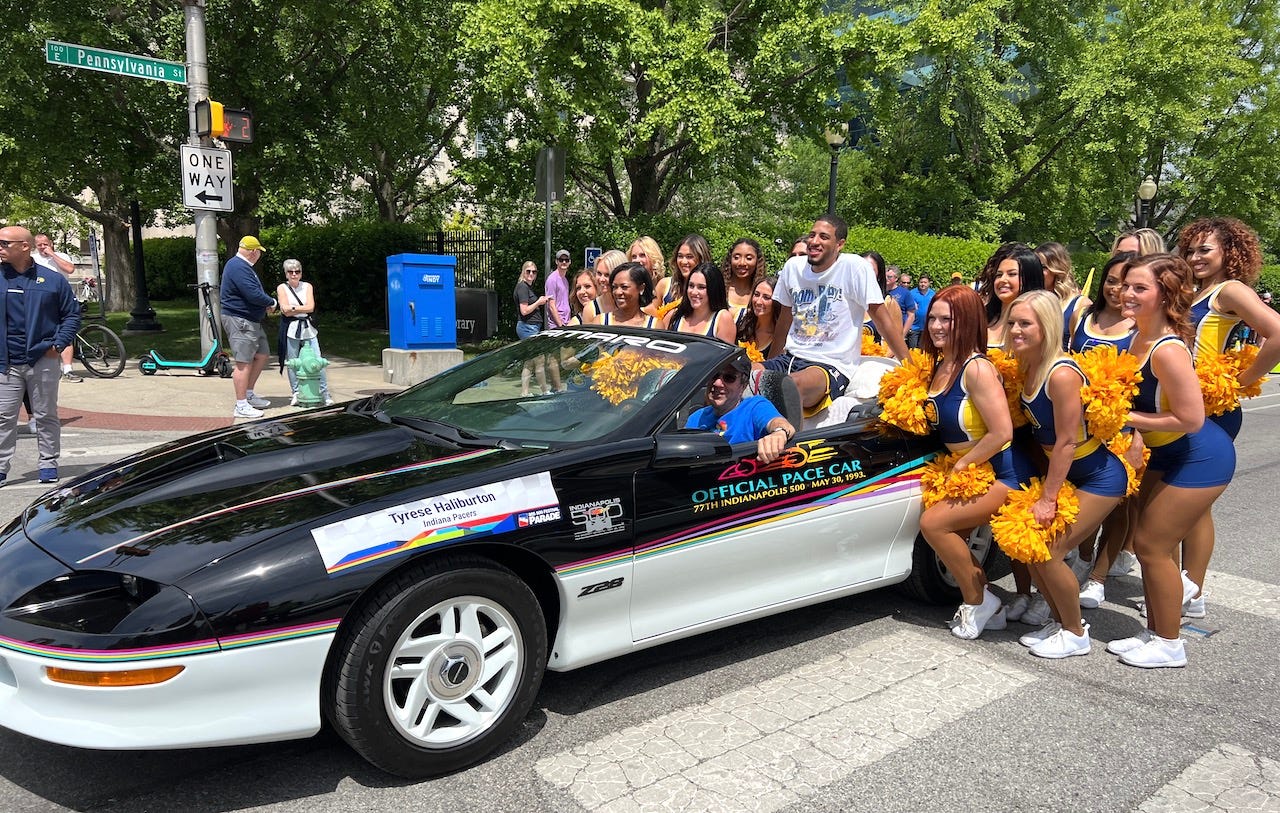This detailed photograph captures a moment at an intersection on Pennsylvania Street, marked by a street lamp and a traffic crosswalk signal, during a parade. At the center of the image is a distinctive black and white convertible Chevrolet Camaro, prominently labeled as the official Pace Car for the 77th Indianapolis 500 on May 30th, 1993. The car's driver, wearing a black baseball cap, sunglasses, and a blue t-shirt, has his left arm casually hanging out of the convertible. A notable figure, likely a celebrity or athlete, stands in the back of the car, smiling broadly.

Surrounding the car is a vibrant group of cheerleaders, approximately 24 in number, donning blue and yellow uniforms with golden pom-poms. They are posing enthusiastically around the car and the celebrity, suggesting a photograph being taken by an off-scene photographer. The festive scene is further enhanced by the presence of passers-by, a scooter leaning on the nearby lamppost, and someone on a bicycle at the left edge of the photograph. A security guard is also visible, ensuring the event proceeds without disturbances. The overall atmosphere conveys a celebratory pep rally or parade, with the intersection serving as a temporary stage for this picturesque moment.